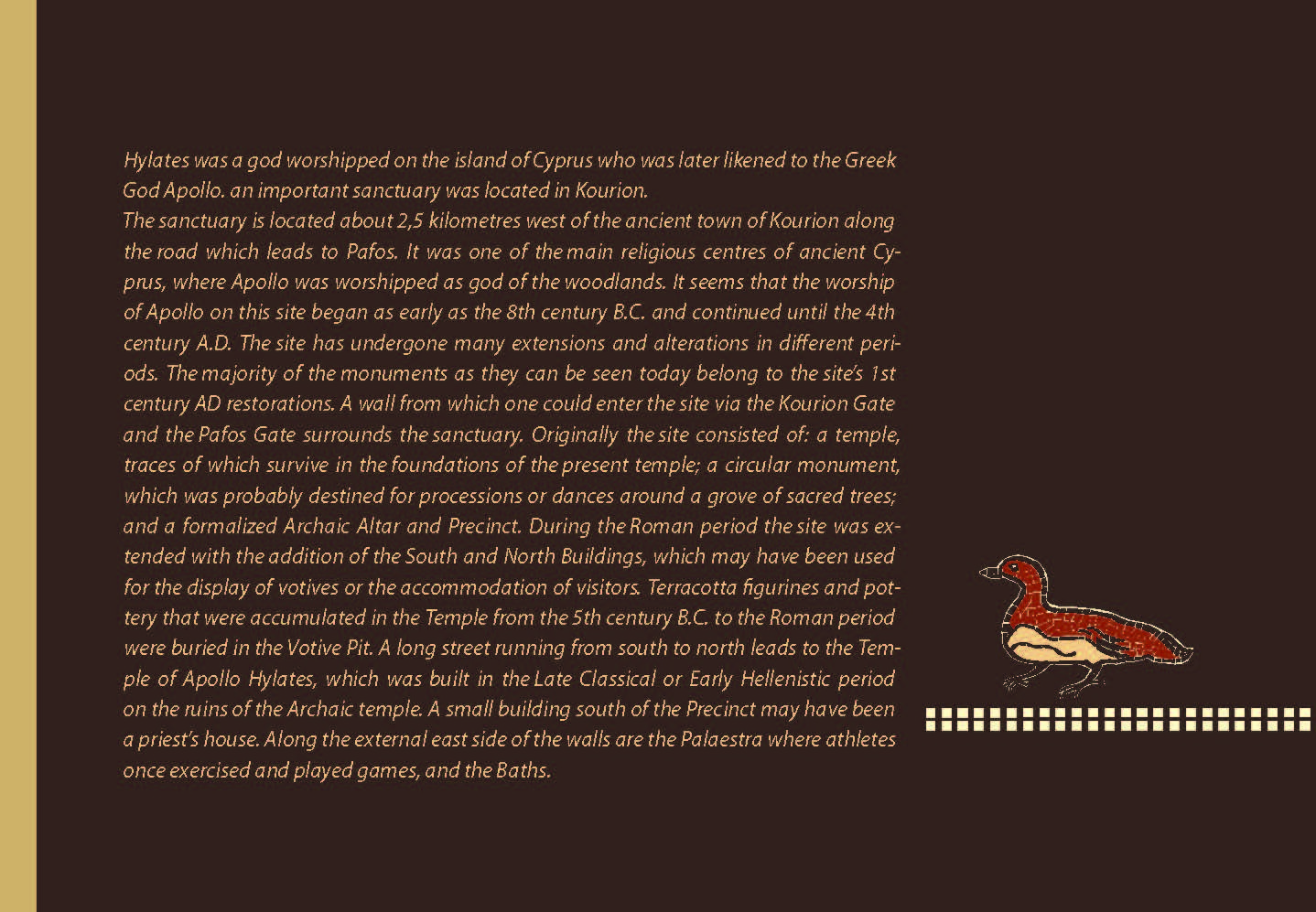This image features an informational placard with a brown background and black text providing a detailed historical account. It explains that Hylates, worshipped on Cyprus, was later likened to the Greek god Apollo. An important sanctuary located around 2.5 km west of the ancient town of Corion along the road to Paphos was one of ancient Cyprus's main religious centers. Here, Apollo was venerated as the woodland deity from the 8th century BC to the 4th century AD. The site saw various extensions and alterations, and most monuments visible today date back to the 1st century AD restorations. Notable components included an early temple foundation, a circular monument for rituals, a formal archaic altar, and buildings added during the Roman period for votive displays and visitor accommodations. Artifacts such as terracotta figurines and pottery from the 5th century BC to the Roman era were buried in the votive pit. The temple of Apollo Hylates, rebuilt in the late classical or early Hellenistic period, stood along a long street running south to north. Additional structures included a possible priest's house and an outdoor palaestra next to the external eastern walls. On the right side of the placard, there is a small depiction of a red duck with a tan belly walking across a digital-looking boardwalk, adding an unusual, whimsical touch to the historical information.